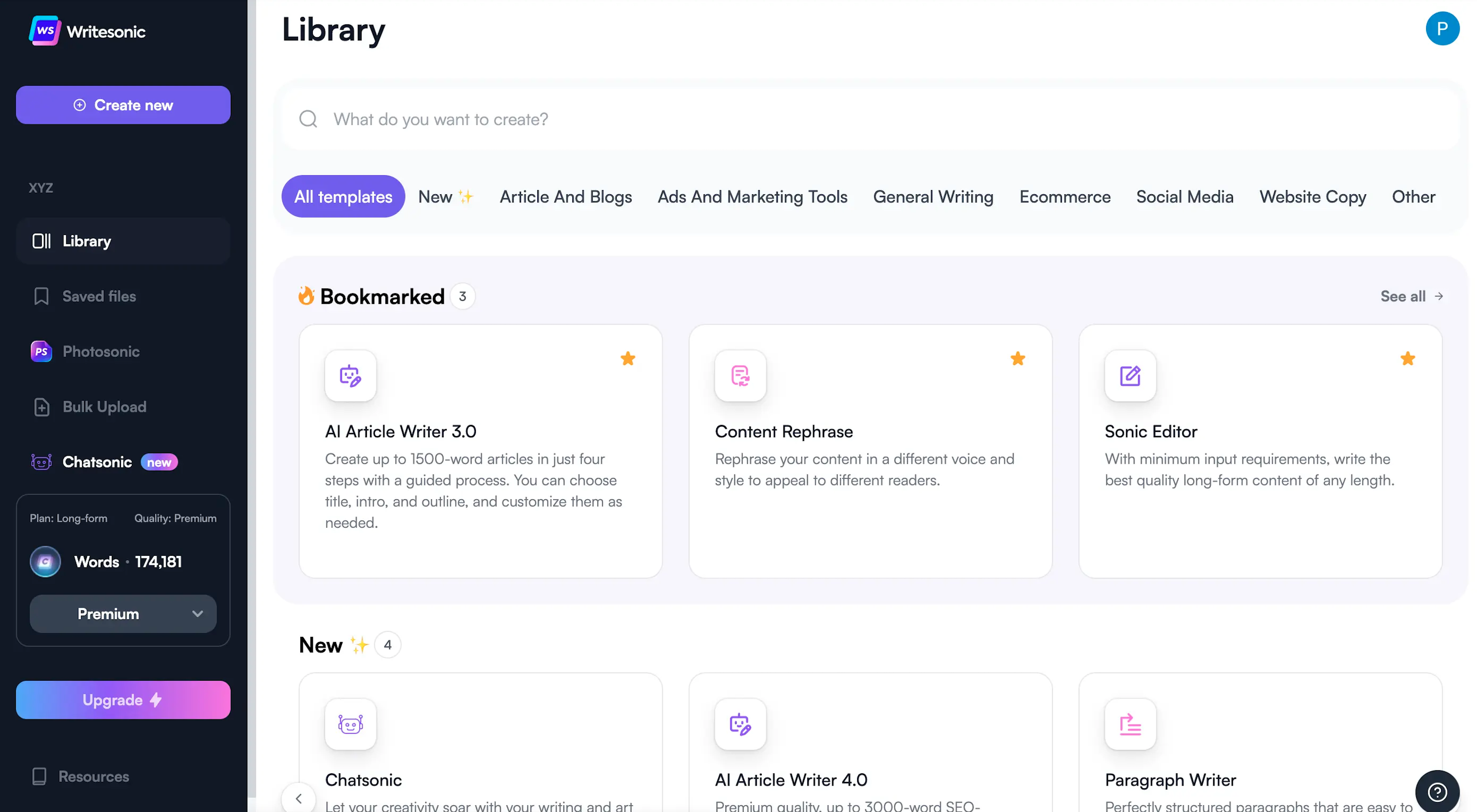This is a detailed screenshot of a computer interface likely displaying a content creation tool or platform. 

On the left side of the screen, there is a black column with various navigation elements. The top section of this column features a neon blue and pink rectangular box with the letters "WS" in the middle. To the right of this box, you'll find the label "Right Sonic" prominently displayed. Below this label, there is a purple button labeled "Create Now."

Moving towards the central part of the screen, the left column highlights the 'Library' option, indicating that this section is currently active. The right side of the screen has a white background with black text. At the top, it features the heading "Library." Directly beneath the heading, there is a search bar with the placeholder text, "What do you want to create?"

Below the search bar, a row of categories is listed horizontally: "All Templates," "New," "Article and Blogs," "Ads and Marketing Tools," "General Writing," "E-commerce," "Social Media," "Website Copy," and "Other." The "All Templates" category is highlighted within a purple oval-shaped bubble.

Further down, there is a gray rectangular section titled "Bookmarked," featuring three white boxes. These boxes are labeled "AI Article Writer 3.0," "Content Rephrase," and "Sonic Editor."

Beneath the bookmarked section, there is another section titled "New," containing three boxes. These are labeled "Chat Sonic," "AI Article Writer 4.0," and "Paragraph Writer." 

Overall, the interface is well-organized and categorized, aiding users in navigating through various content creation tools.